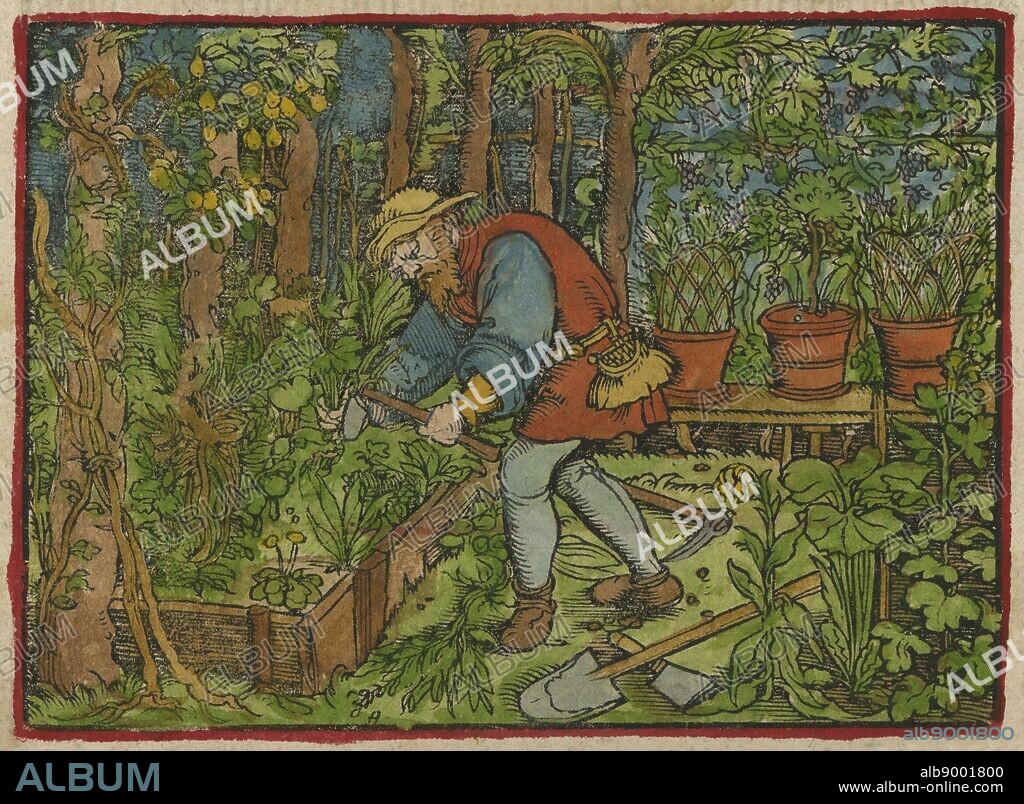This is a detailed, color illustration resembling a watercolor painting set in an outdoor garden scene. At the center of the image is a man with a light brown beard and mustache, notably adorned in a yellow, old-style brimmed hat, reminiscent of medieval or Old English attire. His clothing comprises a red vest, cinched at the waist with a gold belt, which holds a bag for seeds or tools, and features a skirt-like extension. He wears a blue long-sleeved shirt with large puffy sleeves that are rolled up to his elbows, long gray leggings, and brown shoes.

The man is bent over a raised wooden garden bed, grasping a green plant with his right hand while holding a gardening tool with his left. Beside him, lying on the ground are a pickaxe with a long wooden handle and a shovel. Surrounding the main subject, the outdoor setting is lush with several trees, including what appears to be a lemon tree to the left and various potted plants and vines towards the top right. The image features a watermark labeled "album" throughout, with the same text prominent in the bottom left corner and a website mark in the bottom right corner.